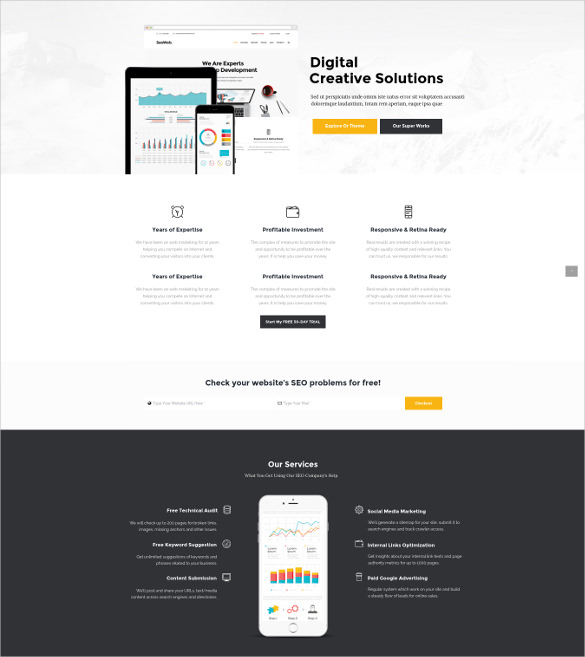Certainly! Here’s a detailed, cleaned-up caption for the image described:

---

The image design is split into distinct sections. The top two-thirds showcases a clean white background featuring digital device representations: the top of a web browser, a tablet displaying a web page, and a smartphone with statistical data. A backdrop of outlined mountains adds depth to the design. Text within this section reads "We are experts in development," accompanied by a laptop illustration. To the right, bold black text spells out "Digital Creative Solutions" (DCS), followed by additional details. A gold bar with white text and a black bar with white text are positioned below.

The middle section continues the white background theme and presents six bullet points arranged in two rows of three. Each point includes an icon and descriptive text:
1. A clock icon with "Years of Expertise" and accompanying text.
2. A wallet icon with "Profitable Investment" and accompanying text.
3. A chip icon with "Responsive and Ready" and accompanying text.
Repeating the icons, the second row reemphasizes "Years of Expertise," "Profitable Investment," and "Responsive and Ready" with corresponding text. Below these points, a black label with white text states, "Check your website's SEO problems for free," flanked by images and relevant text. Central to this section, images and more in-depth content enrich the message, culminating in a gold box with white text on the right.

The bottom third transitions to a black background, prominently featuring "Our Services" in white text, followed by detailed information. This section is organized into two columns of three bullet points each, flanking an image of an iPhone displaying bar and line graphs:
- The left column features three icons (a cylinder, a circle, a square) with white titles and accompanying text.
- The right column mirrors this with three different icons (a round icon, a square icon, and a cylinder icon) also labelled with white titles and descriptive text.

---